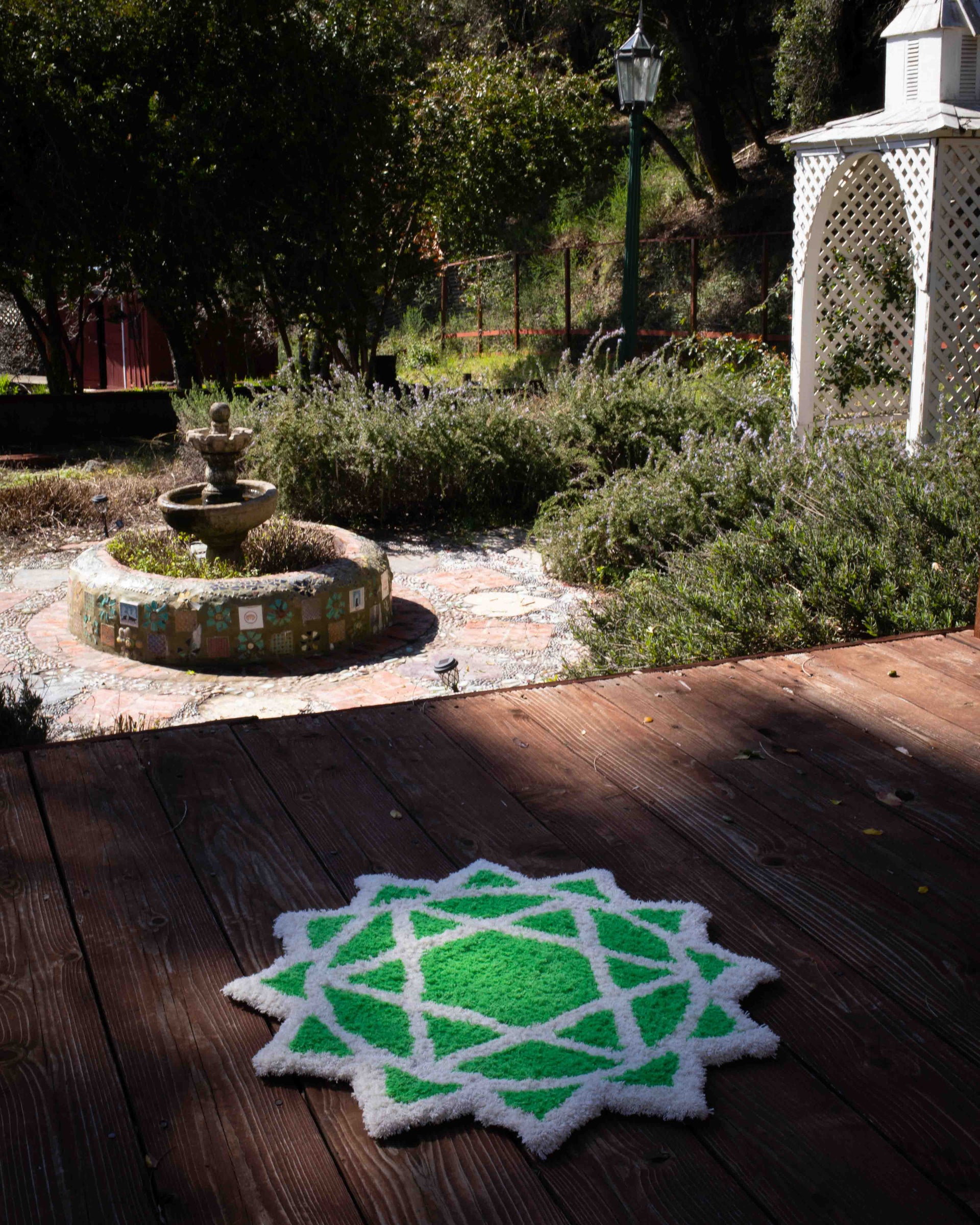This photograph captures a detailed scene of a backyard viewed from a wooden deck with a reddish stain. Prominently featured on the deck is a white rug with green accents, displaying a Star of David at its center. To the right, a white gazebo adorned with lush green plants adds charm to the garden. There is a non-functional rock water fountain with a circular design, surrounded by tiles and a central bowl, now overgrown with weeds. A trellis structure with a small rooftop stands nearby, suggesting an entryway to the garden. A residential-style lamp resembling a lantern is also visible, and in the background, a hill covered with trees and rocks rises, adding a natural backdrop to this eclectic outdoor space.